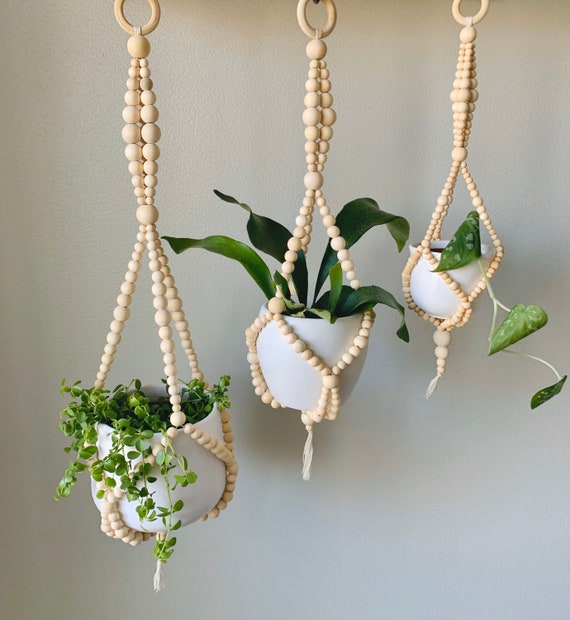The image is a color photograph in portrait orientation, showcasing three white hanging plant containers, each with a green plant inside. They are arranged in a descending diagonal from the lower left to the upper right. The containers are suspended from intricate macrame-style holders made of natural light-wood beads, creating a visually appealing composition against a white wall.

Each beaded hanger consists of three strands that fan out to securely wrap around the containers. The pattern of the beads varies slightly in size, adding texture and depth to the design. The strands converge midway down each hanger around a larger bead, before splitting out again to cradle the pots. The macrame holders are attached to a partially cropped round ring at the top of the image.

The leftmost plant container hangs the lowest and supports a lush, ivy-like green plant that drapes elegantly over its sides. The central container is at a medium height, housing long, dark green leaves reminiscent of palm fronds. The rightmost and highest container holds a plant with larger, vine-like leaves.

The photographic style is representational realism, capturing the details and textures of the materials and plants with clarity and precision.